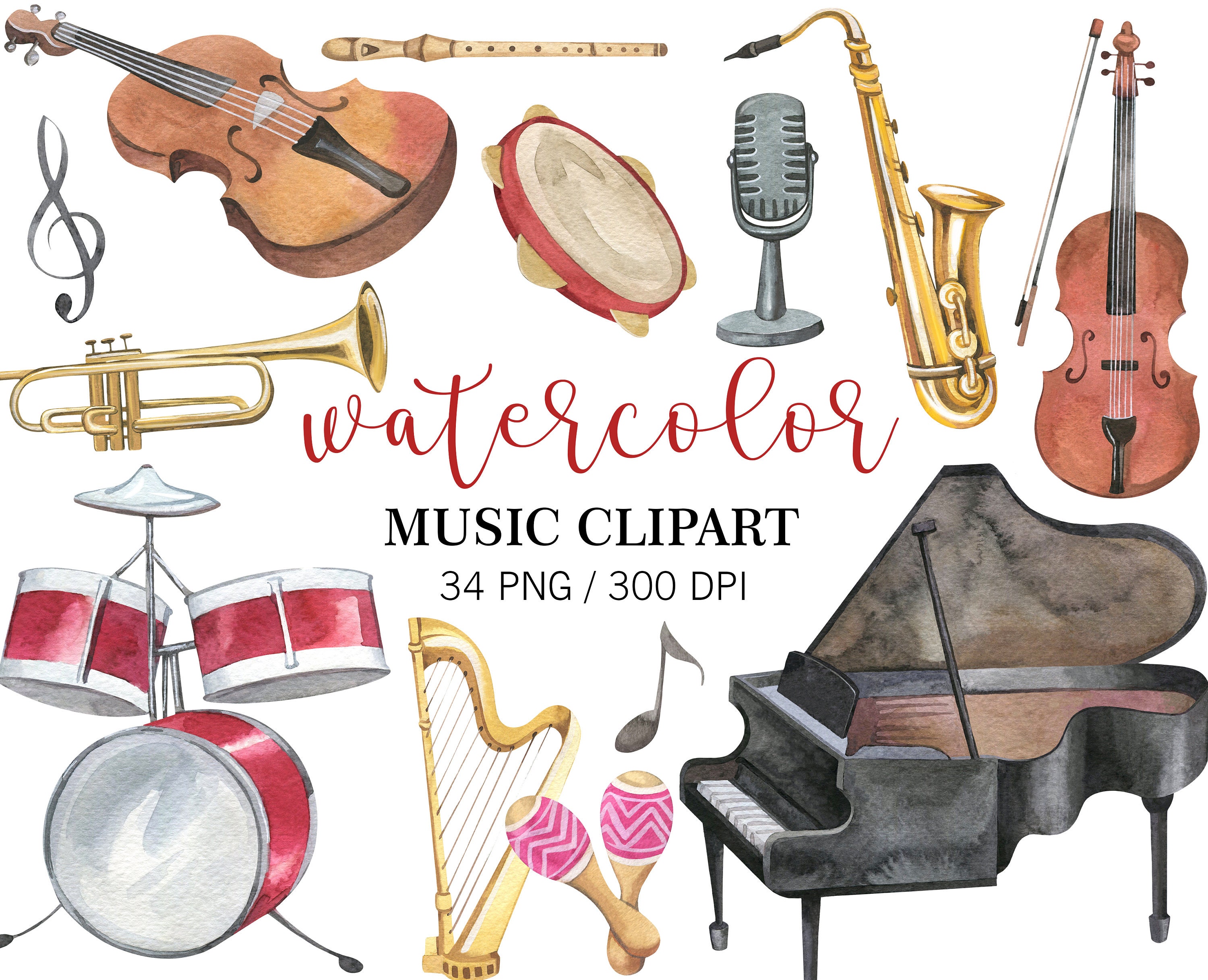This image features a vibrant collection of hand-drawn musical instruments, arranged in a collage-like style with careful attention to detail. In the upper left-hand corner, there's a brown string instrument, which could either be a violin or cello. Below this, there's a musical clef symbol, and to the right of that is a yellow recorder (or possibly a flute). Adjacent to the recorder is a red-ringed tambourine with a tan hide.

To the right of the tambourine is a silver old-fashioned microphone, followed by a gold saxophone. Continuing to the right, there's another string instrument, likely a violin. To the left and below the cello, there's a trumpet, and underneath that, a detailed red and white drum set.

Next to the drum set is a harp, and to the right of the harp are a pair of maracas. Above the maracas is a musical note symbol. Nearby, in the lower right corner, there's a black grand piano. 
In the very center of the composition, the text "watercolor" is written in cursive red. Directly below it, in black uppercase letters, it says "MUSIC CLIPART," followed by "34 PNG / 300 DPI" in black. The mix of both familiar and unique instruments highlights the diversity and liveliness of musical expression.